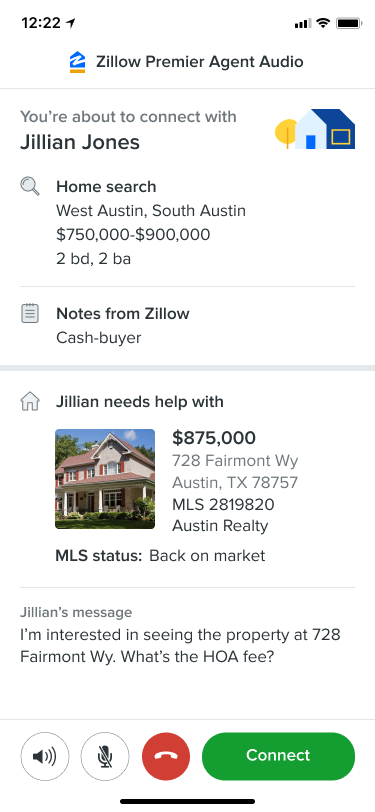This mobile web view of the Zillow Premier Agent Audio contact page features a highly detailed display of both interface and contextual information. 

At the top, the status bar indicates the current time as 12:22, accompanied by three out of four cell signal strength bars highlighted in black, with the fourth bar in gray. The Wi-Fi strength is full, depicted in black, and the phone’s battery icon is entirely filled in black, signifying a full charge.

The interface begins with the Zillow logo, beneath which is an orange bar and the text "Zillow Premier Agent Audio". A thin gray separator follows, displaying the message "You are about to connect with Jillian Jones," alongside a whimsical clip-art of a house with a bluish facade and a yellow-orange tree.

Further down is a search section featuring a magnifying glass icon and the text "Home Search," with details about the West Austin and South Austin areas. The price range for listed homes is displayed as $750,000 to $900,000, specifying options for two bedrooms and two baths. Beside this, a notes icon introduces notes from Zillow Cash Buyer.

A thicker horizontal gray line separates this from the next section, which features a home icon and the text "Jillian Helps With," adjacent to the image of an actual two-story home. This home has red shutters, grayish siding, and a porch. Its listed price is $750,000, with the address 728 Fairmont Way, Austin TX 7875, and MLS number 2819 820 from Austin Realty. The MLS status indicates the home is "Back on the Market."

Jillian's message is prominently displayed, reading "I'm interested in seeing the property at this address, what's the HOA fee?"

The bottom of the screen contains action buttons, including an audio button, a microphone toggle, an end call button in red with a white phone icon, and a green, oval-shaped connect button with white text reading "Connect." A black horizontal line spans the bottom of the page, visually marking the end of this thorough and interactive mobile web interface.